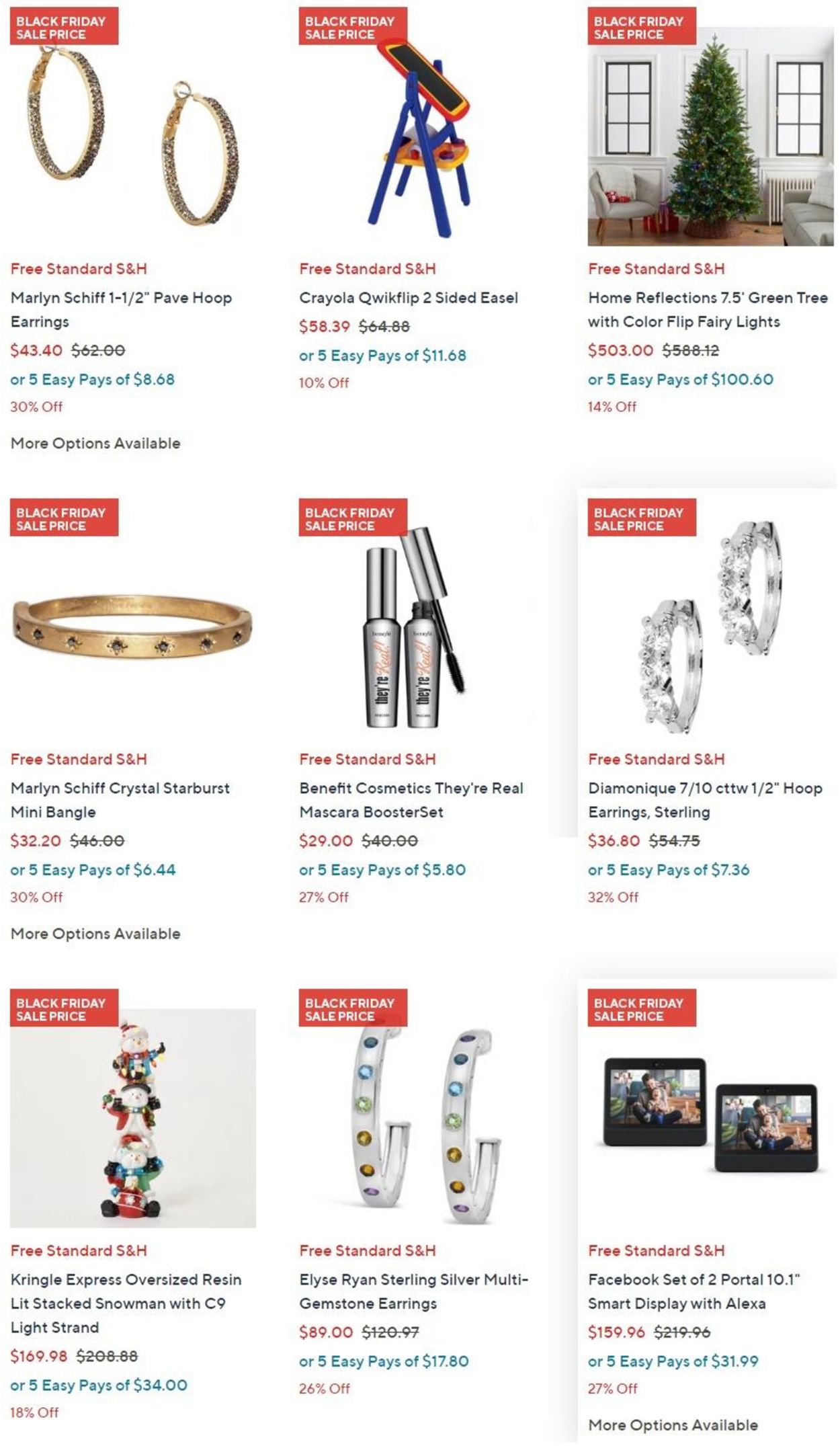This screenshot features a webpage from an e-commerce site advertising a variety of items for sale, with a strong focus on holiday-themed products. The site is clearly gearing up for Black Friday, as indicated by a prominent banner and red tags stating "Black Friday Sale" next to each item. 

Among the highlighted items, there are hoop earrings, gemstone earrings, and other types of jewelry. There is also a Crayola Quick Flip 2-Sided Easel for children, likely appealing as a holiday gift. The seasonal offerings include an artificial Christmas tree, adorned with colorful decorations, and a set of Kris Kringle Express oversized snowmen priced at $169. In total, the page displays nine different items.

The overall theme suggests a festive shopping experience with significant discounts, capturing the holiday shopping spirit and preparing customers for the upcoming festivities. There is no specific company branding visible on the screenshot, but it appears to cater to both traditional Black Friday shoppers and those looking for online deals, possibly indicating promotions for Cyber Monday as well.